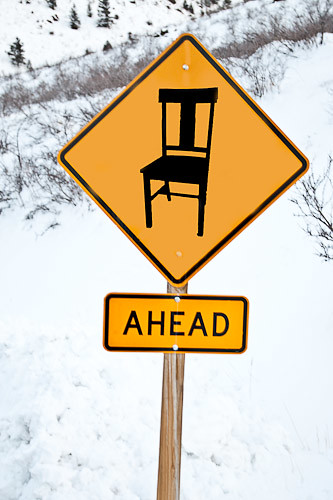Captured in the great outdoors, this image features a serene snow-covered mountain as the backdrop. The glistening white snow contrasts beautifully with the sprigs of resilient green trees poking through, along with several bushes showing signs of winter dormancy with their bare branches. Dominating the foreground, a prominent yellow, diamond-shaped sign is affixed to a sturdy wooden pole with silver nails. The sign features a black pictogram of a chair, commonly indicating a chairlift ahead. Directly beneath it, an attached yellow rectangular sign bears the clear, black inscription "AHEAD," guiding adventurers toward their next destination.